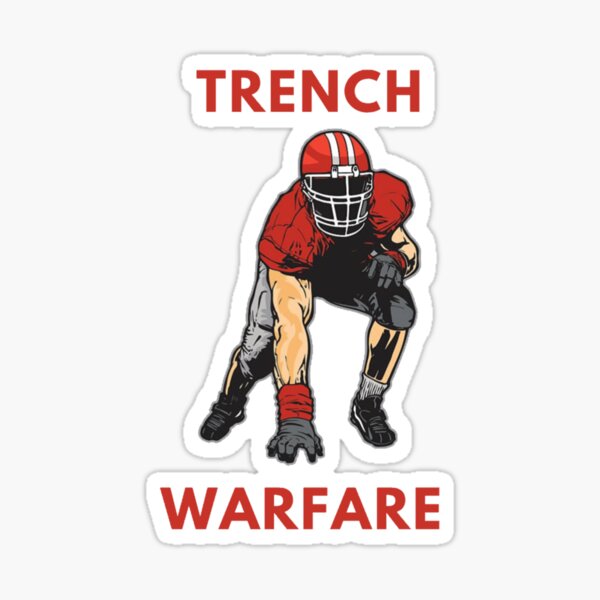This image features a cutout magnet or sticker displayed against a plain white background. At the center of the design is a crouching football player positioned to face the viewer directly. The upper part of the image is adorned with the word "TRENCH" in bold, red capital letters, while the bottom features the word "WARFARE," equally bold and in red capital letters. The football player is depicted in an athletic stance, with one gray-gloved hand touching the unseen ground beneath him. His bared arms and lower legs are visible, emphasizing his physical readiness. 

The player is outfitted in gray padded pants and a red shirt equipped with shoulder pads, adding to his robust appearance. His helmet, which sports red and white stripes, features a black void in place of a visible face, giving the figure an anonymous, intense presence. The contrast of colors and the dynamic stance effectively convey the intensity and readiness associated with trench warfare in football.